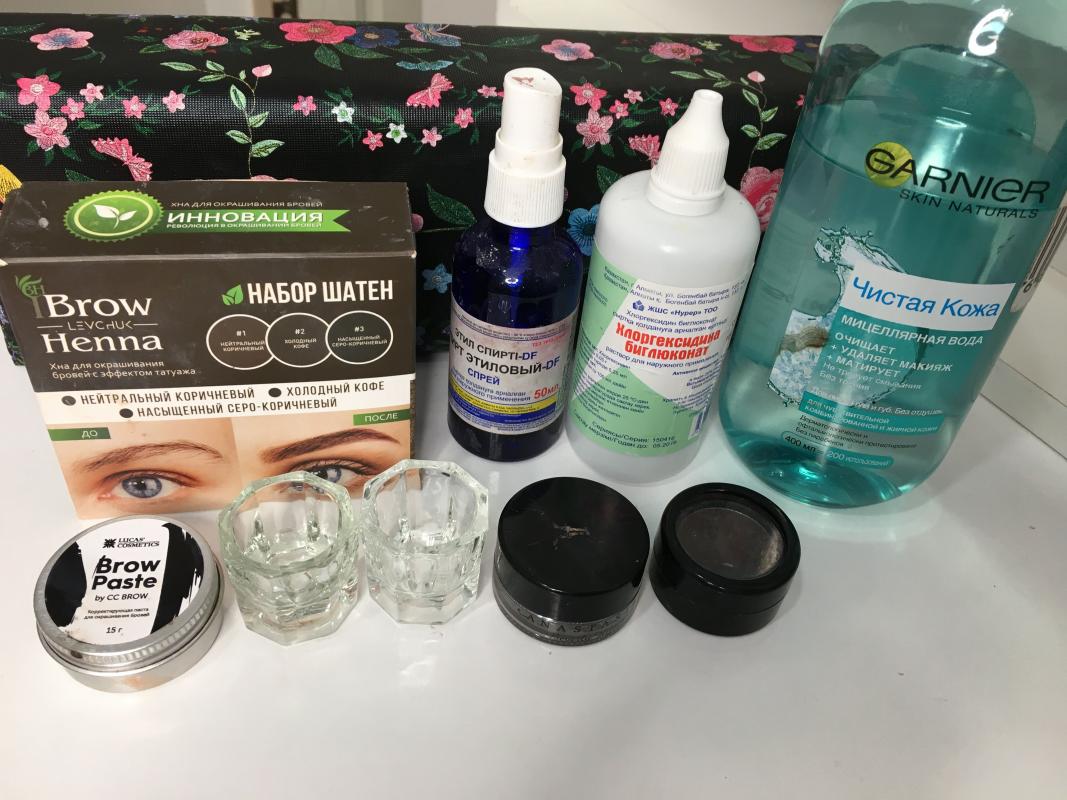A neatly organized white countertop adjacent to a matching white wall. At the far back, partially obscured by the background, sits a fashionably designed makeup bag adorned with a black base and intricate patterns of pink and purple flowers accompanied by green leaves. To the far right, a teal bottle labeled "Garnier" contains clear liquid, with text in a foreign language, possibly Russian. Moving left, there lies a white bottle with a green label, likely contact lens solution, and further left, a blue bottle with a blue and yellow label, also marked with non-English text, perhaps Russian. Next to it stands a brown box with green labeling titled "Brow Henna," featuring an image of blue eyes showcasing the product. In front of the box sits a small container of brow paste. Additionally, two small round containers for contact lenses appear nearby. Completing the arrangement, two black round containers are positioned on the left side, adding to the assortment of personal care items.